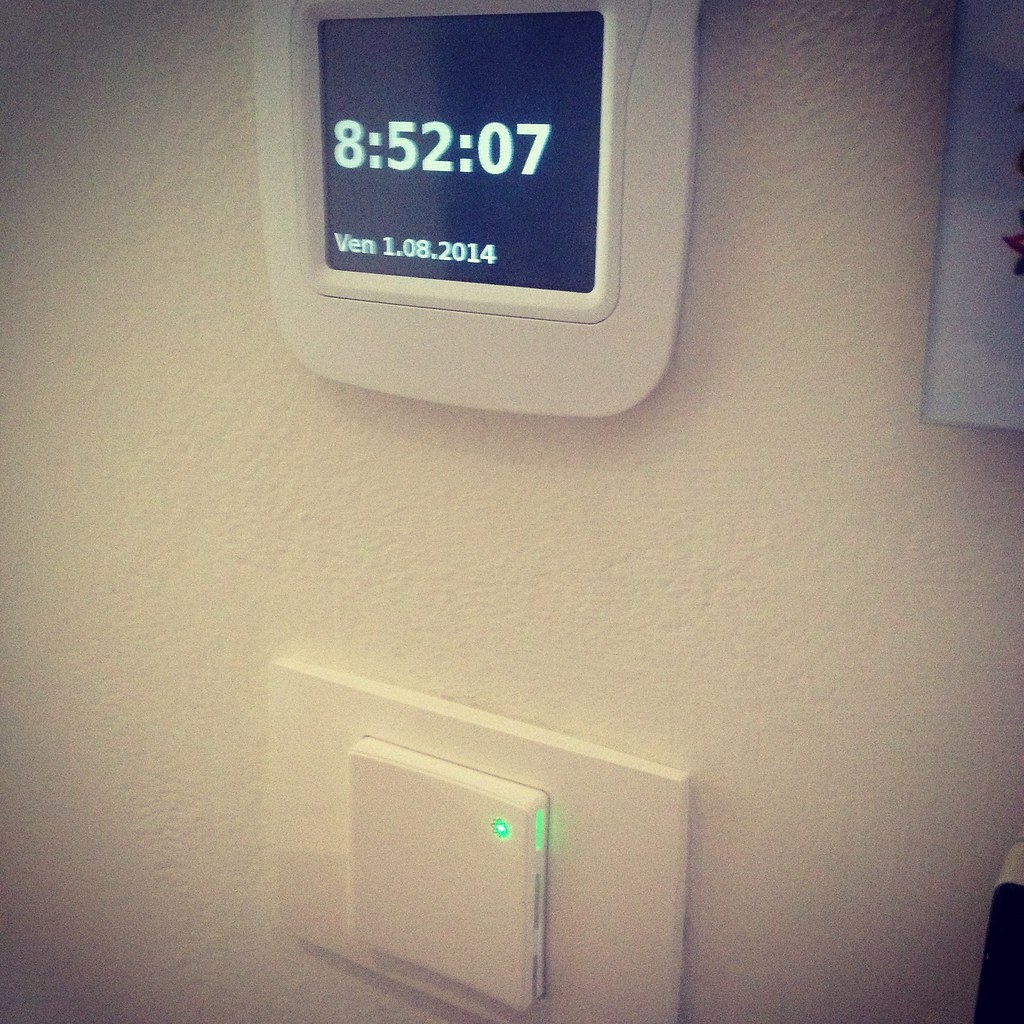A close-up view of a white wall features two notable devices. At the top, a smart home monitor is affixed to the wall, displaying the current time as 8:52:07 and the date as "VEN 1.08.2014," indicating "Vendredi" or "Friday" in French. The monitor has a black background with white lettering, providing a stark contrast that enhances readability. Below, a smart plug is inserted into an electrical outlet. This plug emanates a green illumination and is equipped with multiple USB ports, indicating its advanced, multifunctional nature. Other than these two devices, the wall is bare, emphasizing the focus on the smart home technology.